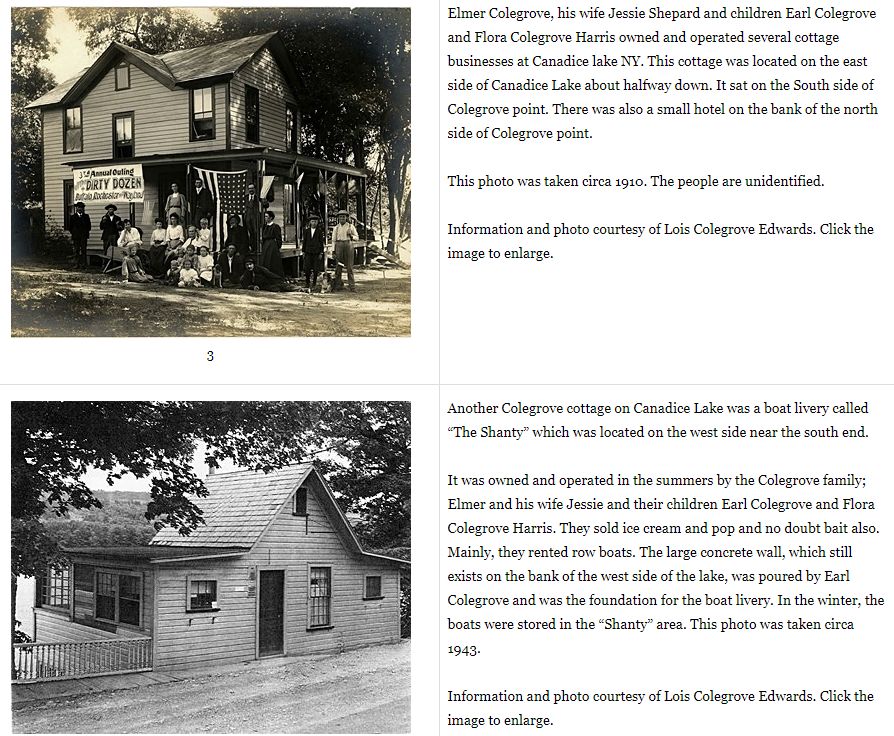This information display features historical photographs and details about heritage buildings operated by the Colgrove family at Canadis Lake, New York. The display is divided into four quadrants, with each quadrant featuring either a photograph or accompanying text. 

The top left quadrant showcases a sepia-toned photograph from 1910, depicting a group of people sitting and standing around the porch of a two-story turn-of-the-century frame house. This house is identified as the Colgrove Cottage, a significant property for the Colgrove family, who were known for operating several cottage businesses in the area. The people in the photo remain unidentified. Adjacent to this image, the top right quadrant contains the descriptive text explaining the historical context of the Colgrove Cottage and its association with the family's business activities at Canadis Lake.

The bottom left quadrant features another vintage photograph, also possibly in sepia or black and white. This image portrays a different Colgrove cottage named "The Shanty," which functioned as a boat livery situated on the lake's west side near the south. This cottage, owned and operated by the Colgrove family, was a popular spot where visitors could rent rowboats and purchase ice cream during the summer. The adjacent bottom right quadrant provides detailed text on "The Shanty," further elucidating its role and significance within the Colgrove family's entrepreneurial endeavors. 

Overall, the display captures the essence of early 20th-century life and commerce at Canadis Lake, highlighting the Colgrove family's contributions to the local heritage.